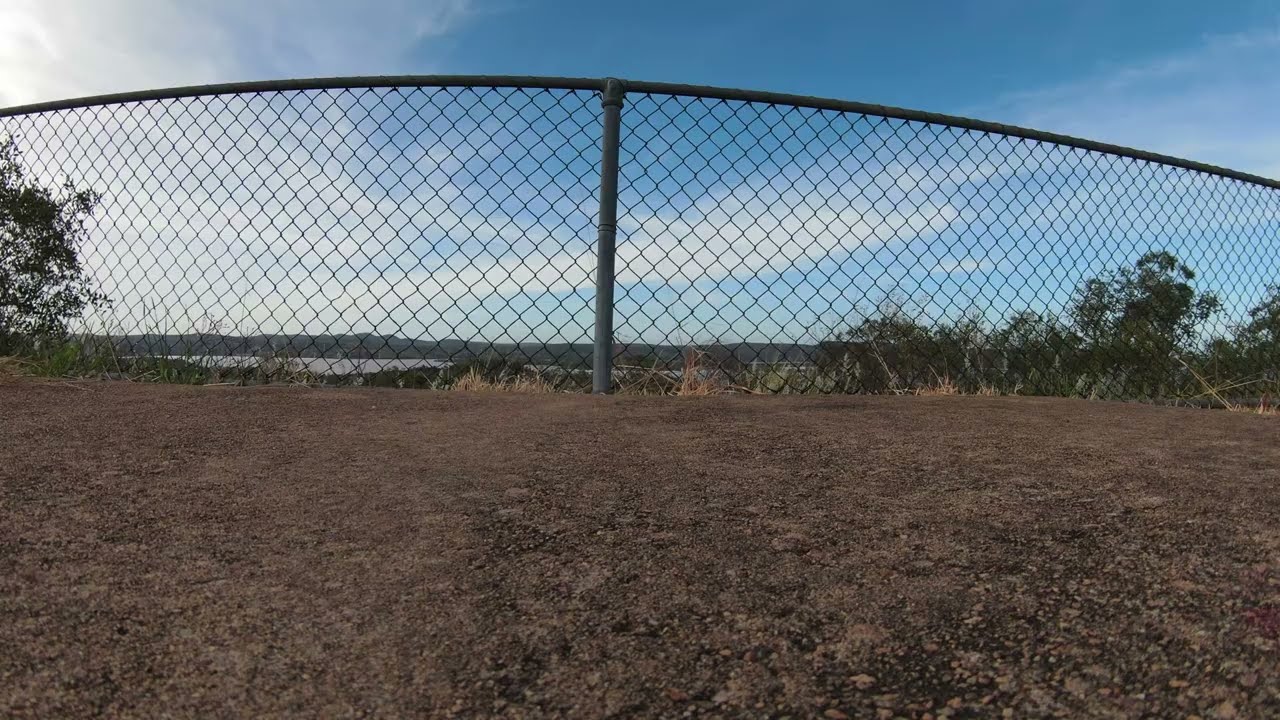The photograph, taken from ground level on a partly cloudy day, captures the barren expanse of a dirt field dominating the lower half of the image. The ground, devoid of grass or weeds, appears stark and rugged. In the center, a metal pole or fence post supports a chain-link fence that seemingly curves inward at the top left before extending outward through the top right of the frame. The fence, patterned in a diamond shape, dips slightly in the middle, adding to the impression of curvature. 

Beyond the fence, one can see a mixture of thin trees or bushes and patches of grass, mostly dead but with hints of green, climbing up along the fence. The background features a sloped landscape heading downhill, revealing a further-off view of rooftops and hilly terrain. Subtly, the distant horizon reveals mountains under a blue sky dotted with wispy clouds. The backdrop also includes a tree line forming on both the left and right edges of the image, framing the scene and emphasizing the natural, slightly untamed setting.